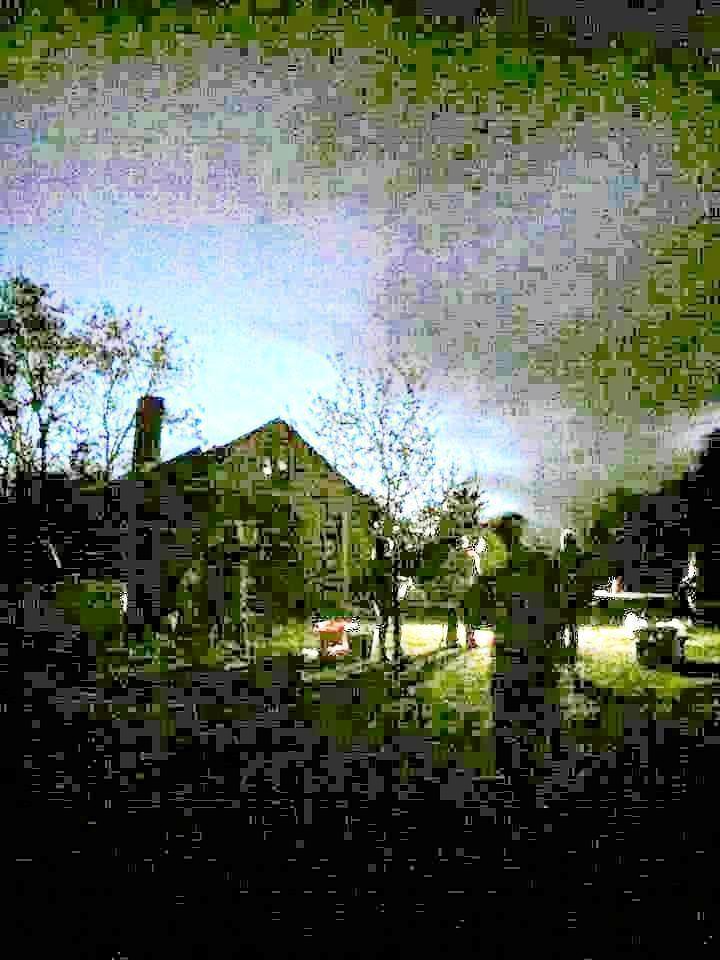The image is a highly pixelated and blurred photograph, predominantly green at the top and bottom with a mix of gray, blue, and black elements. The focal point seems to be a farmhouse, identifiable by its chimney, with sparse trees scattered around. Several figures, anywhere from three to four, are standing in the yard, casting shadows due to a light source that might be coming from the sky or possibly a bonfire. The figures and the house appear in shades of gray and black, adding to the overall pixelated effect. The sky is somewhat blue and purple, transitioning to gray and black as it moves up the image. The bottom of the picture is darker, blending from black to green and gray, making it challenging to discern specific details.